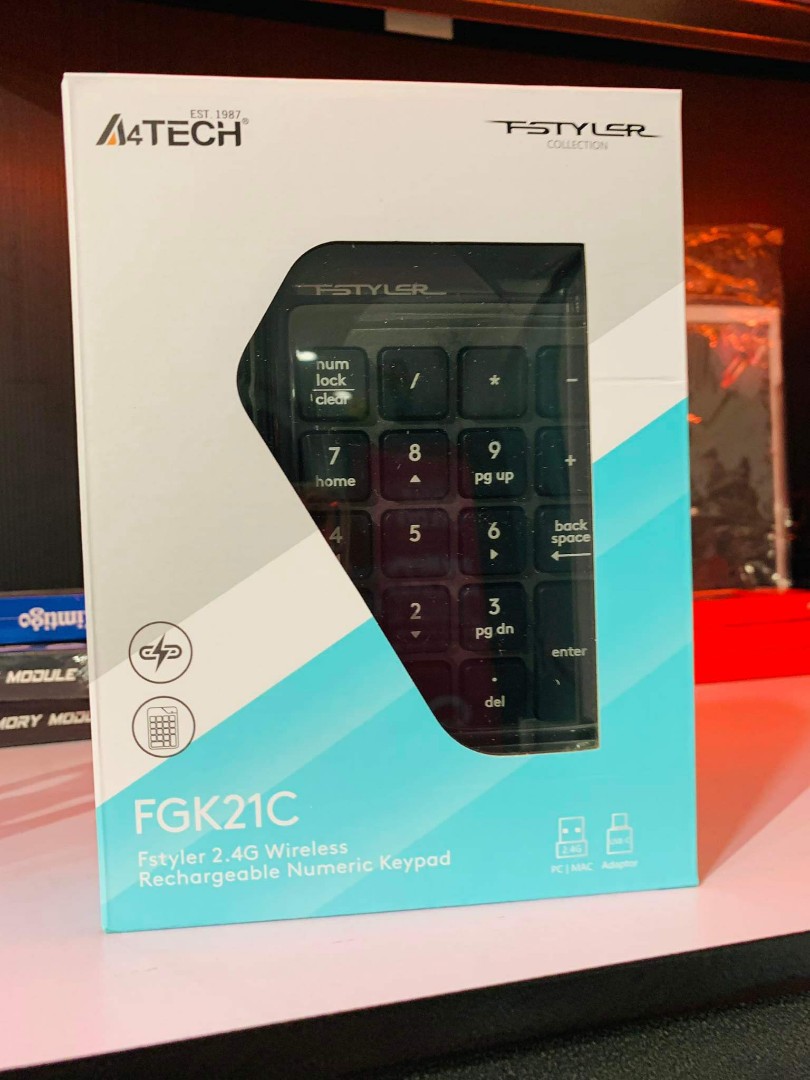This product photo features an A4 Tech wireless numeric keypad, still encased in its original packaging. The small, square box stands upright at the edge of a pristine white table, starkly contrasting with the minimalist backdrop. Located at the top left corner of the box, the A4 Tech logo prominently displays the brand, while to the right, "FS Styler" is emblazoned in a sleek, futuristic font. A clear cutout on the front of the box allows a glimpse of the keypad inside. The keypad itself is compact and black, with a number lock key at the top left, followed by keys for forward slash, asterisk, and minus, alongside the numerical keys. An enter button is positioned on the bottom right of the keypad. Across the top of the box, "FS Styler" is reiterated. At the bottom of the box, the model number FGK21C is provided, alongside the description "FS Styler 2.4G Wireless Rechargeable Numeric Pad," accompanied by a USB icon for connectivity indication.